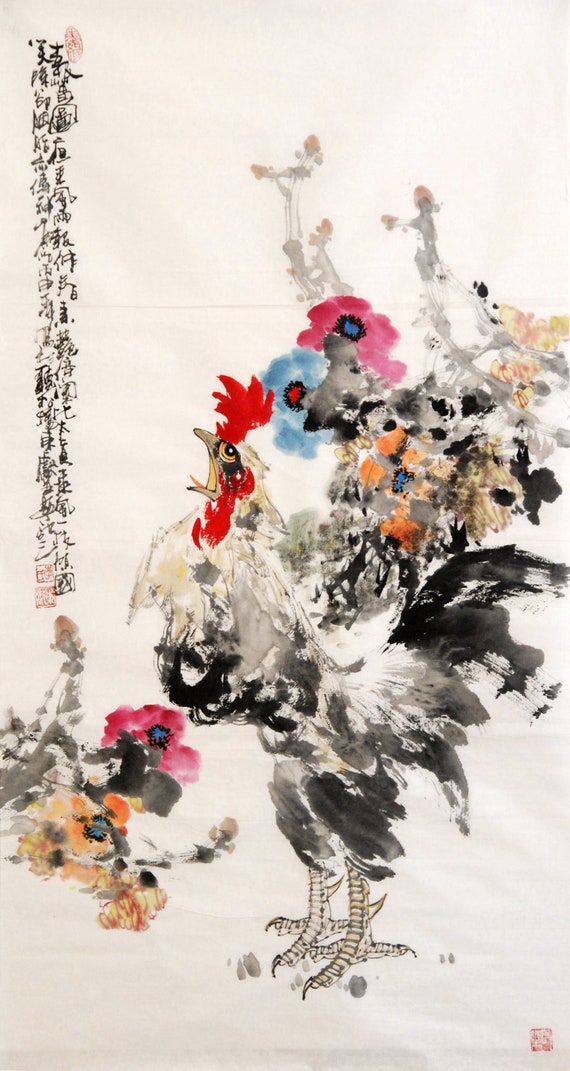This image depicts a traditional East Asian, likely Chinese, piece of artwork that is rectangular in shape with a vertical, portrait orientation, approximately three times as tall as it is wide. It features a predominantly off-white background. Along the left side of the image, from the top left corner down to just over halfway, is a vertical column of Chinese characters, suggestive of a classic ink-and-wash painting style. Below this text, near the lower left section, there are renderings of delicate flowers with varying colors, such as pink with blue and black centers, and orange petals blending into shades of gray.

The centerpiece of the artwork is a vividly detailed rooster situated in the central lower part of the image. The rooster appears to be crowing, with its head and neck arched back. The rooster's plumage is primarily white with nuanced gray feathering, enhanced by black ink outlines adding definition. Its bright red comb and detailed eye, featuring a mix of orange and black hues, stand out strikingly, and the rooster’s open beak even reveals an orange tongue. Behind the rooster are more flower renderings, blending seamlessly with its feathers but distinguishable with pink, light blue, red, and black, adding a touch of color and depth.

At the very bottom right corner of the image is a red rectangular stamp, likely the artist's personal seal, inscribed with characters that are difficult to discern clearly due to their intricate design. The overall composition reflects a harmonious blend of natural elements and calligraphy, characteristic of traditional Chinese art.